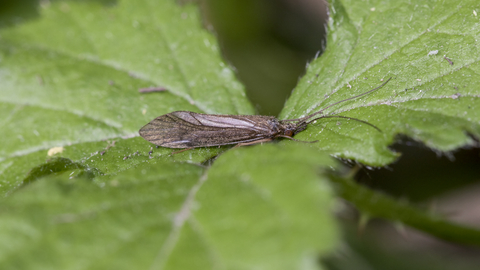A highly detailed, professional close-up photograph captures a scene centered around a leaf that occupies nearly the entire frame. Resting on this large green leaf, which also shows elements of dirt and debris, is a brown insect positioned centrally, possibly a moth, butterfly, or fly. The insect's profile reveals long antennae and a narrow, elongated body with large wings, one of which is prominently visible. Its head is oriented towards the right side of the image. The background is deliberately blurred, drawing sharp focus to the insect and the leaf. The green leaf includes a hint of a stem with thorns visible on the right side, contributing to the natural setting. The photograph, taken in landscape format, emphasizes the insect's delicate details and the textures of the leaf, making it a striking and focused composition.